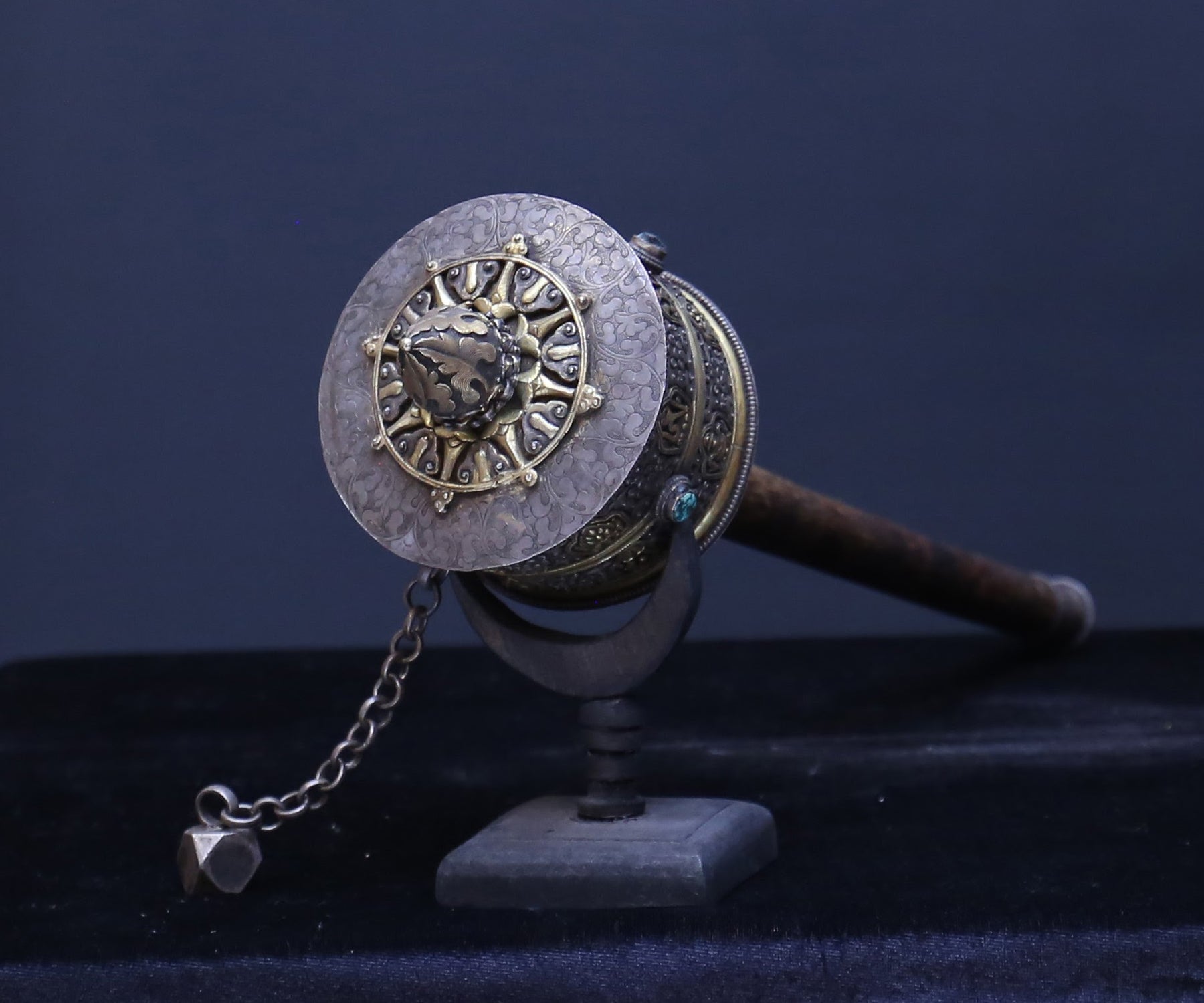The image depicts an intricately designed medieval weapon, resembling a scepter that could be associated with royalty. The weapon features a long, wooden handle extending into the background, becoming blurry as the focus remains on the metallic head. The head of the weapon is cylindrical, finished in silver with intricate floral and leaf designs, and accentuated with gold highlights. A striking feature includes blue jewels positioned near the top and bottom of the cylinder. The top of the weapon culminates in a pointed, crown-like structure, topped with a silver ball. 

This detailed piece rests on a small, stone-like pedestal with the base having a crescent-shaped support. The weapon is further secured by a chain, attaching it to a screw on a black surface. The dark blue to dark purplish background enhances the object's elaborate and high-class appearance, suggesting it might belong to a rich or royal individual. The overall aesthetics suggest it to be more than just a mere weapon; it has the grandeur and refinement befitting a ceremonial or symbolic artifact.